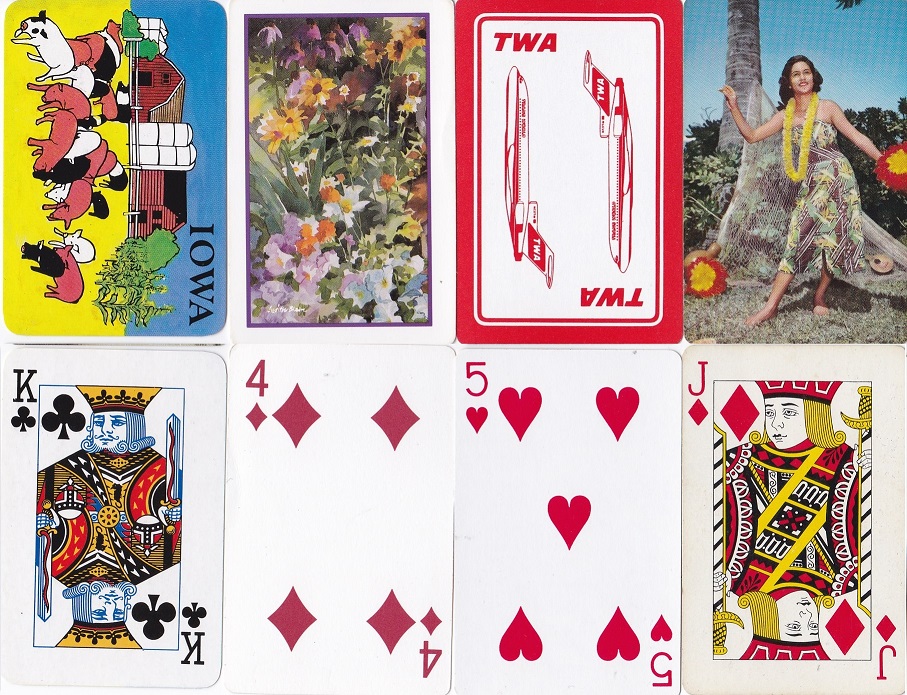The image is divided into two rows, each comprising four images. 

On the bottom row, from left to right:
1. The King of Clubs playing card.
2. The Four of Diamonds playing card.
3. The Five of Hearts playing card.
4. The Jack of Diamonds playing card.

On the top row, from left to right:
1. A postcard oriented on its right side. It features the word "Iowa" in the lower right corner and depicts several cartoon pigs, a red barn, silos, and a yellow ground. The sky is blue but is situated on the right due to the postcard's orientation.
2. A card richly adorned with drawings of flowers in muted hues such as yellow, purple, pale green, and sage green.
3. A TWA card with a red border and white interior. "TWA" is written in red along with two vertical planes—one pointing up and one pointing down. The "TWA" text in the lower right corner is upside down.
4. A postcard showcasing a woman in traditional Hawaiian attire. She is wearing a yellow lei and appears to be performing a hula dance. The background features a blue sky, grass, and a tree trunk.